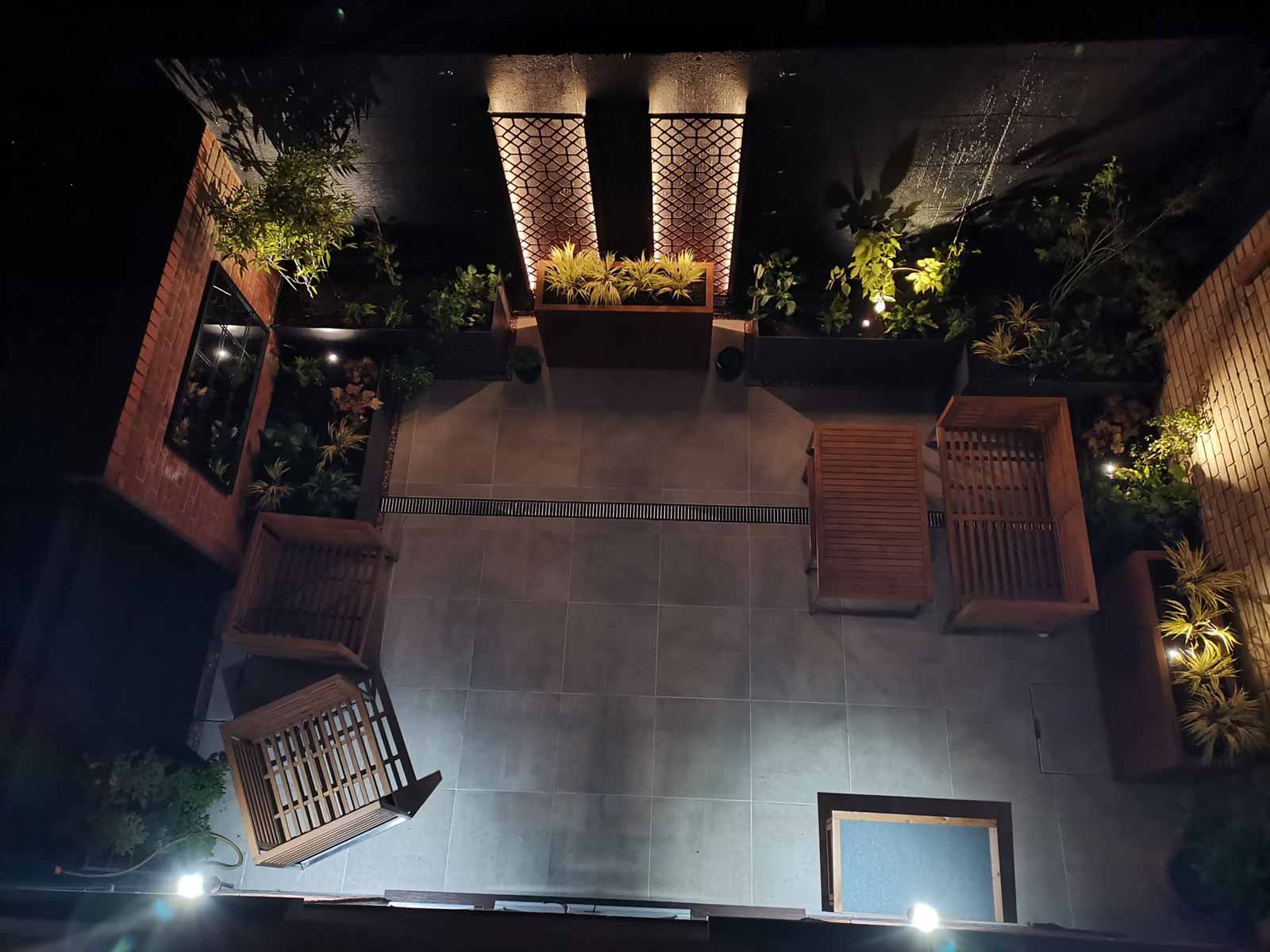This is an aerial photograph of a rectangular, landscaped outdoor patio, possibly taken from a security camera. The patio features large square tiles in varying shades of gray and light brown, creating a modern, elegant flooring. The left side wall is prominently a dark brown brick, adorned with either a window or a mirror with black glass, beneath which are more wooden plant containers hosting lush green and yellow plants. 

At the top center of the courtyard is a wooden flower box with yellow blooms, while additional wooden planters with diverse green foliage line the perimeter on the right and left sides. Scattered across the patio are various pieces of wooden furniture in a cherry wood color. On the bottom left side, two boxy wooden chairs with open slats sit without cushions, offering a minimalist look. On the right side, a similar material loveseat in a darker wood shade stands with a coordinating small table in front.

The back wall features metal tower-like structures housing lights that illuminate the area. String lights from above cast a warm, inviting glow throughout the scene. The right side showcases a beige brick wall with more wooden planters, each with its own light, enhancing the serene ambiance. Overall, the patio is a harmonious blend of nature and modern design, fully equipped for relaxation and outdoor enjoyment.